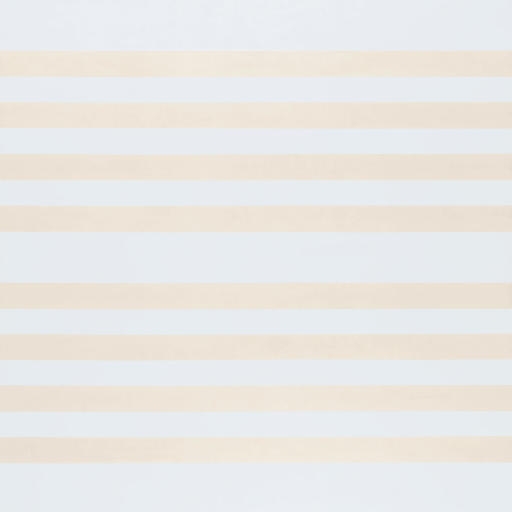The image is a minimalist square with a background gradient that transitions from a darker grayish-blue at the top to a light bluish-white at the bottom. Overlaying this background are eight faint, non-uniform stripes in a pale beige-pink color. These stripes are spaced irregularly across the square, with tighter groupings of four stripes at both the top and bottom of the image and a slightly larger grayish-blue bar in the middle. The overall palette is very light and translucent, creating a subtle blend and the impression of a delicate, almost ethereal pattern.